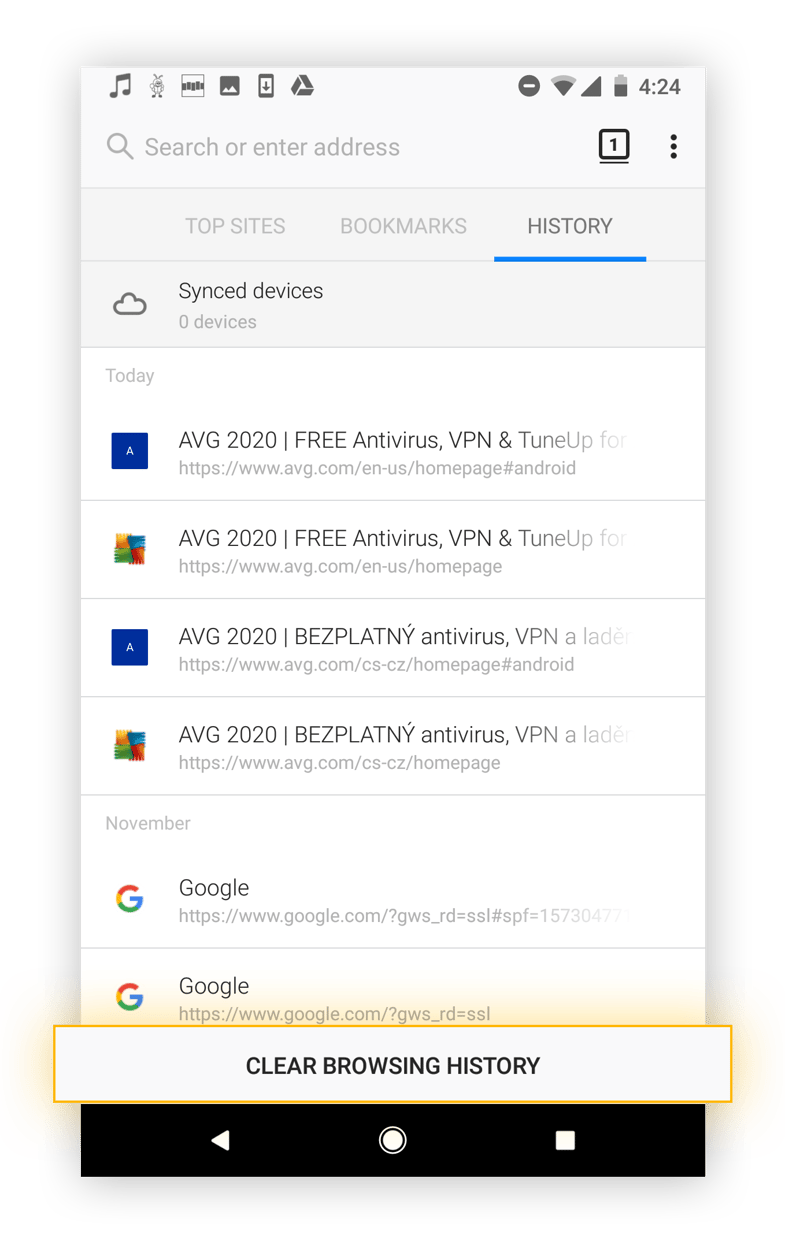The image is a detailed screenshot showcasing the Chrome browsing history on an older Android device. The screenshot itself is bordered by a shadow, creating a distinct frame around it. At the very top of the image, the device's status bar is visible, featuring several grey icons from left to right: a music icon, an insect icon, a multi-line box, a screenshot icon, a download icon in a phone, and a Google Drive logo. These are followed by a 'Do Not Disturb' icon, a WiFi icon, a cellular network icon, a battery icon indicating half charge, and the current time displayed as 4:24, all set against a white background.

Directly below the status bar is a grey text field on a white background, labeled as a search box with the prompt "Search or enter address". Adjacent to this search box is a small square with the number 1 in it and three vertical dots symbolizing a more options menu.

Following this is a segment with a grey background containing three text buttons, labeled "Top sites", "Bookmarks", and "History". The "History" tab is prominently highlighted with darker text and a blue underline. Below this, separated by a thin line, is text reading "Synced devices" accompanied by a cloud icon and the note "zero devices".

The main section of the screenshot features a white background with a small grey header reading "Today", under which multiple website entries are listed. Each entry includes a website logo and titles such as "AVG 2020 free antivirus" or "AVG 2020" in various languages. Lower in the screenshot is a section labeled "November" showing two instances of visits to Google's homepage in the browsing history.

At the bottom of the screenshot, a prominent button with bold black text reading "Clear browsing history" is placed on a white background with a glow-like yellow outline, suggesting it is an interactive element. Finally, the screenshot captures the Android device's black control bar at the bottom, displaying the back, home, and recent app buttons represented by white shapes.